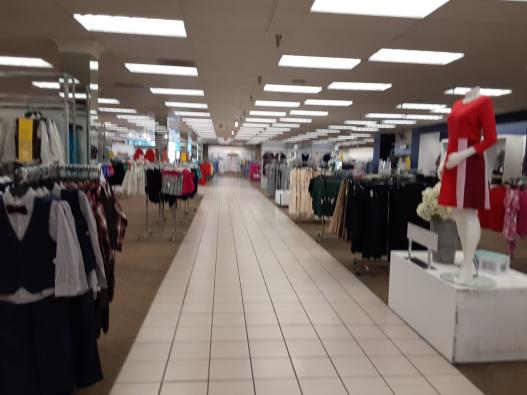The image depicts a spacious aisle inside a department store. The aisle is lined with white stone tiles running centrally down its length, creating a clear path through the store. The ceiling above is light gray and outfitted with large square lights, ensuring the area is well-lit. Notably, there is a sprinkler system lining the ceiling as well.

On the right side of the aisle, the women's clothing section is displayed, with numerous dresses and blouses visible in the background. A prominent feature is a mannequin standing on a large white pedestal, dressed in a striking long-sleeved red dress with a red and white striped skirt. Near the mannequin, there are signs and a large bouquet of flowers in a gray vase, adding a decorative touch to the display.

The left side of the aisle features what appears to be boys' clothing, including outfits with white shirts, vests, and bow-ties, suggestive of formal wear. The overall impression is that of a vast department store, filled with a diverse range of clothing for different demographics, meticulously organized along the expansive aisle.